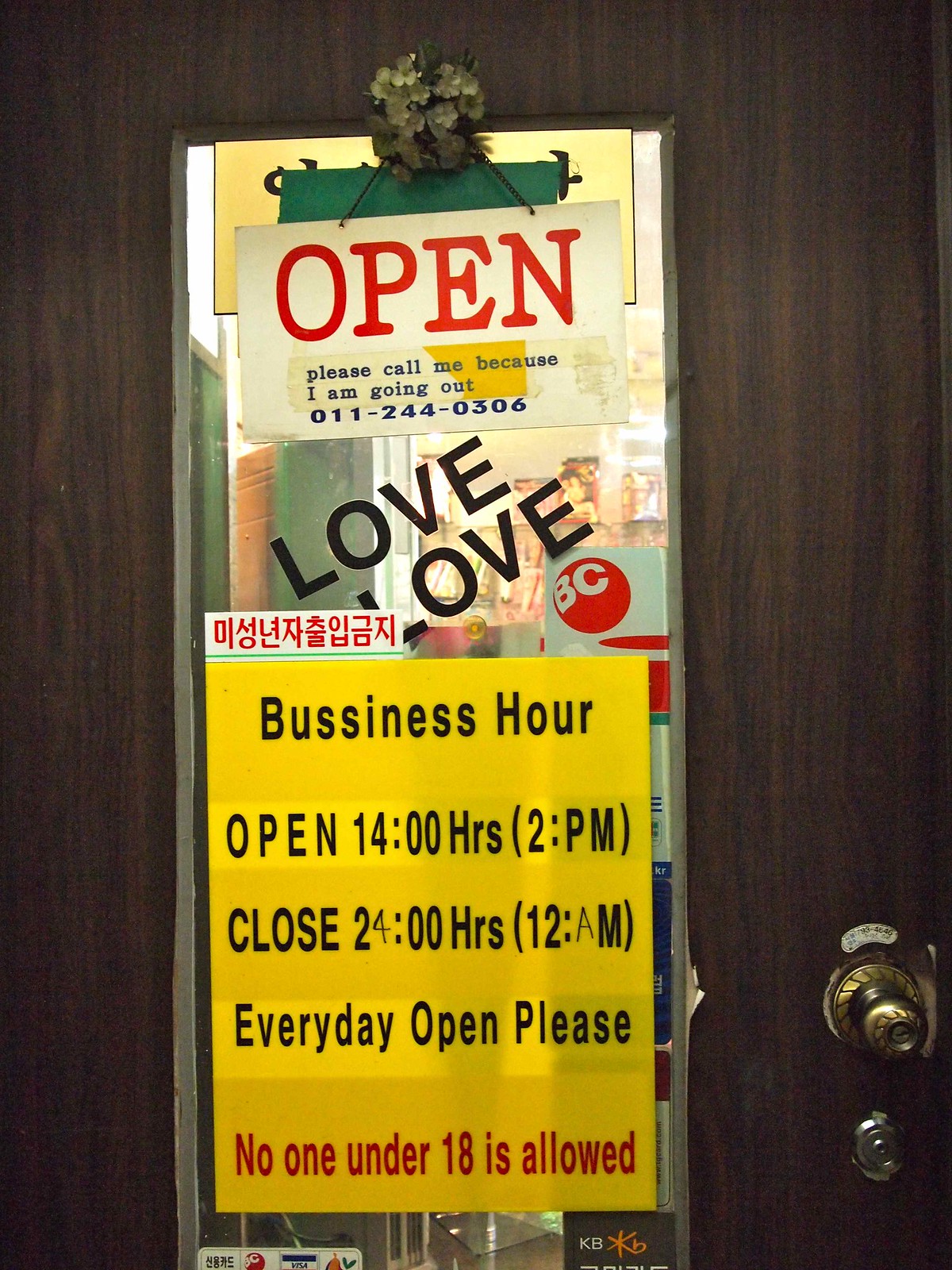The image features a dark, walnut-colored wooden door with a visible wood grain texture. At the lower right corner of the door is a circular gold doorknob with intricate gold wire detailing at its base, and directly below this knob is a silver-colored lock. The door also includes a glass pane, and hanging from it is a white sign with various details. At the top of the sign, in large red capital letters, it reads "OPEN." Beneath this, in dark blue text, it says, "Please call me because I’m going out," followed by the phone number "011-244-0306." Diagonally across the sign is the word "love love" written in black. Toward the bottom left, there is a small white section displaying red Asian characters. Below this, a yellow segment with black text lists the business hours as "Open 14:00 (2 p.m.), Close 24:00 (12 a.m.), Every Day Open Please." The bottom of the sign, in red text, clearly states, "No one under 18 is allowed."